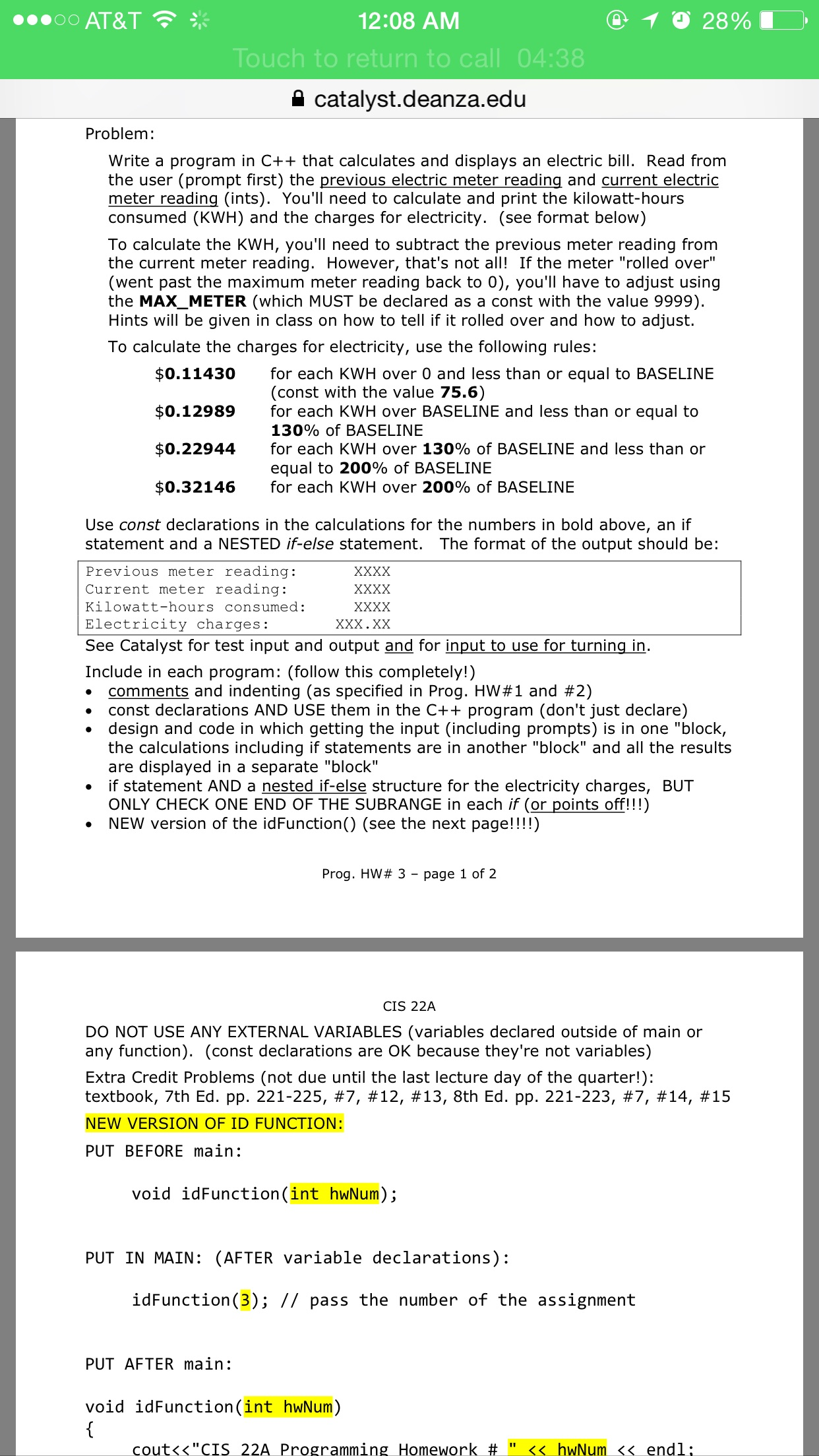This screenshot depicts a detailed programming homework assignment accessed from the Catalyst platform at dinza.edu, displayed on a smartphone screen. The top bar of the phone shows it is 12:08 AM, with the network carrier AT&T, a battery level at 28%, and an ongoing call notification lasting 4 minutes and 38 seconds.

The assignment is for the CIS 22A course and instructs students to develop a C++ program to calculate and display an electric bill. The problem statement provides specific instructions:
1. Prompt the user to enter previous and current electric meter readings, both as integers.
2. Calculate the kilowatt hours used by subtracting the previous reading from the current one.
3. Handle scenarios where the meter has rolled over using the maximum meter value of 9999.
4. Use provided hints for managing the rollover adjustment.

The assignment further details the programming requirements, emphasizing the use of an if statement and a nested if-else structure. The output format must display:
- Previous meter reading
- Current meter reading
- Kilowatt hours consumed
- Electricity charges

Additional guidelines include placing comments, identifying, and structuring code blocks appropriately and following provided examples and comments. The task demands using a new version of the ID function defined as `void function(int HWNUM)`, which must be placed before the main function and invoked after variable declarations within the main function.

For extra credit, students must avoid using any external variables, and specific extra credit problems are referenced in the textbook. 

The document is a comprehensive assignment designed to teach students how to write a C++ program focusing on calculation, conditional structures, and appropriate code documentation.